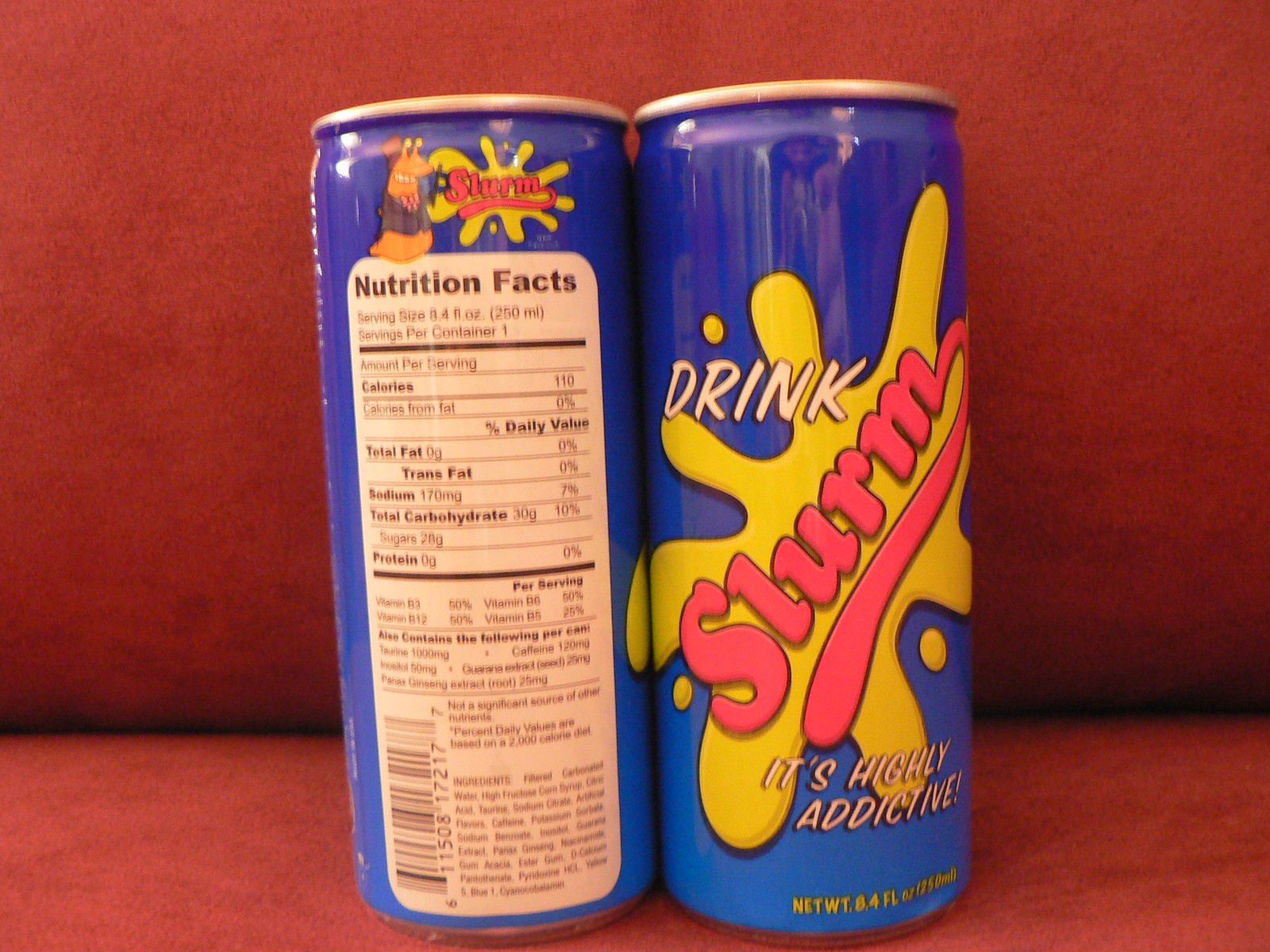In this image, two blue cans are showcased against a completely red backdrop—the floor and the wall are both red. The can on the left is turned to display its back, revealing a white and black nutrition facts panel complete with a UPC code, ingredients, and various nutritional details. Above this panel, a quirky brown slug character, wearing a green vest and hat, adds a whimsical touch to the design. The right can, presented from the front, features a prominent yellow splash graphic with the word "SLURM" in red letters slanted diagonally from lower left to upper right. Additionally, above this splash in white letters, it says "DRINK," and underneath it, "SLURM" followed by "It's highly addictive" in smaller yellow letters. The cans display a slight gradient, being darker at the top and lighter at the bottom, adding depth and intrigue to their blue exteriors.